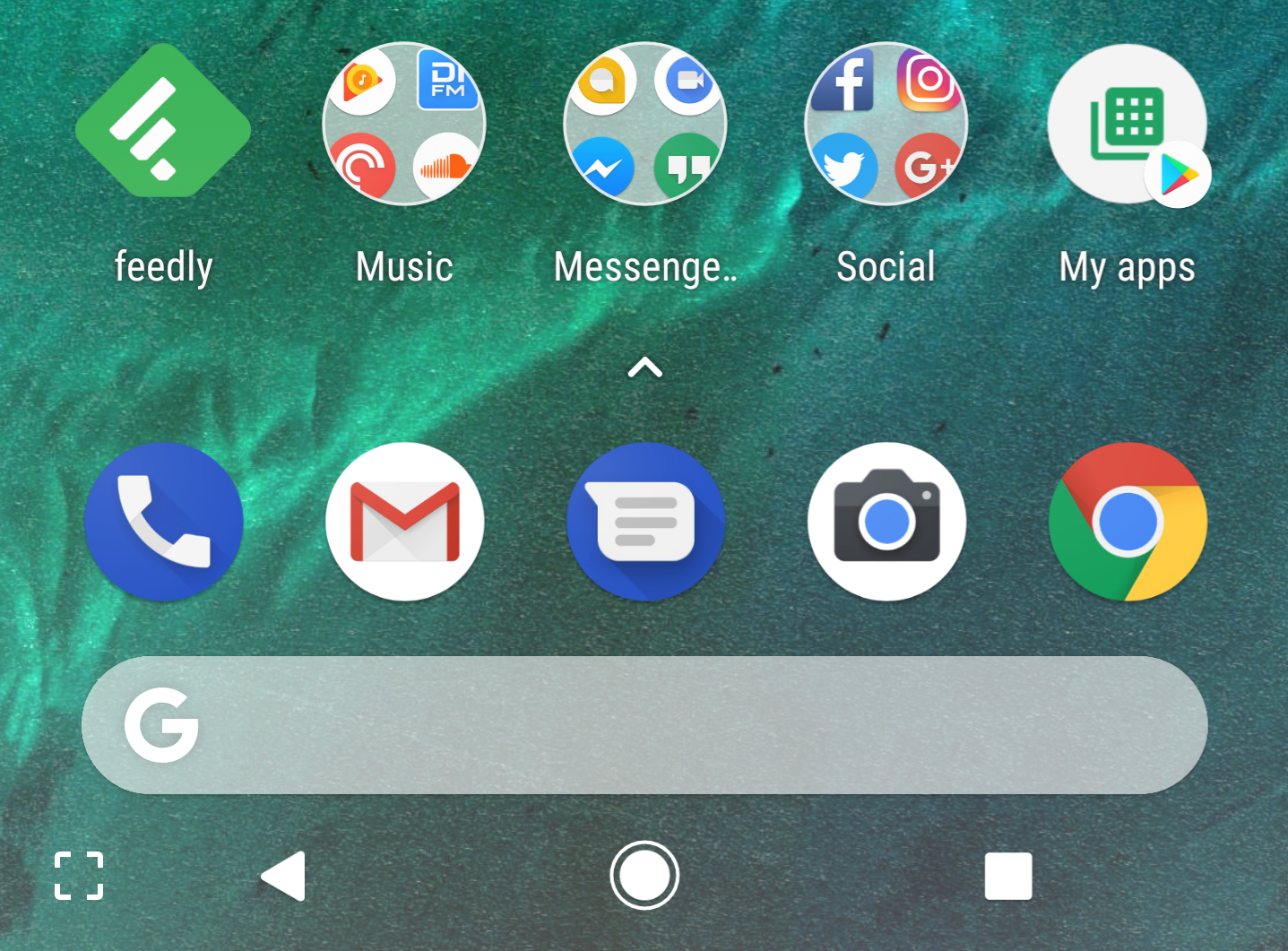This image displays a screenshot of an Android device's home screen. Positioned in the bottom left corner, we see a full-screen button, followed by a backward play button, a filled white circle with an outlined white circle around it, and a pause button. At the top of the screen is a prominent search bar adorned with the Google "G" logo on the left. Below this bar are several app icons: Phone, Contacts, Gmail, Messages, Camera, and Google Chrome. Just above this row, we have an app named Feedly and three distinct app folders labeled as Music, Messenger, and Social. The final item on this line is a folder named My Apps. Within the Music folder, icons for apps like SoundCloud are visible. The Social folder includes app icons for Facebook, Instagram, Twitter, and Google+.